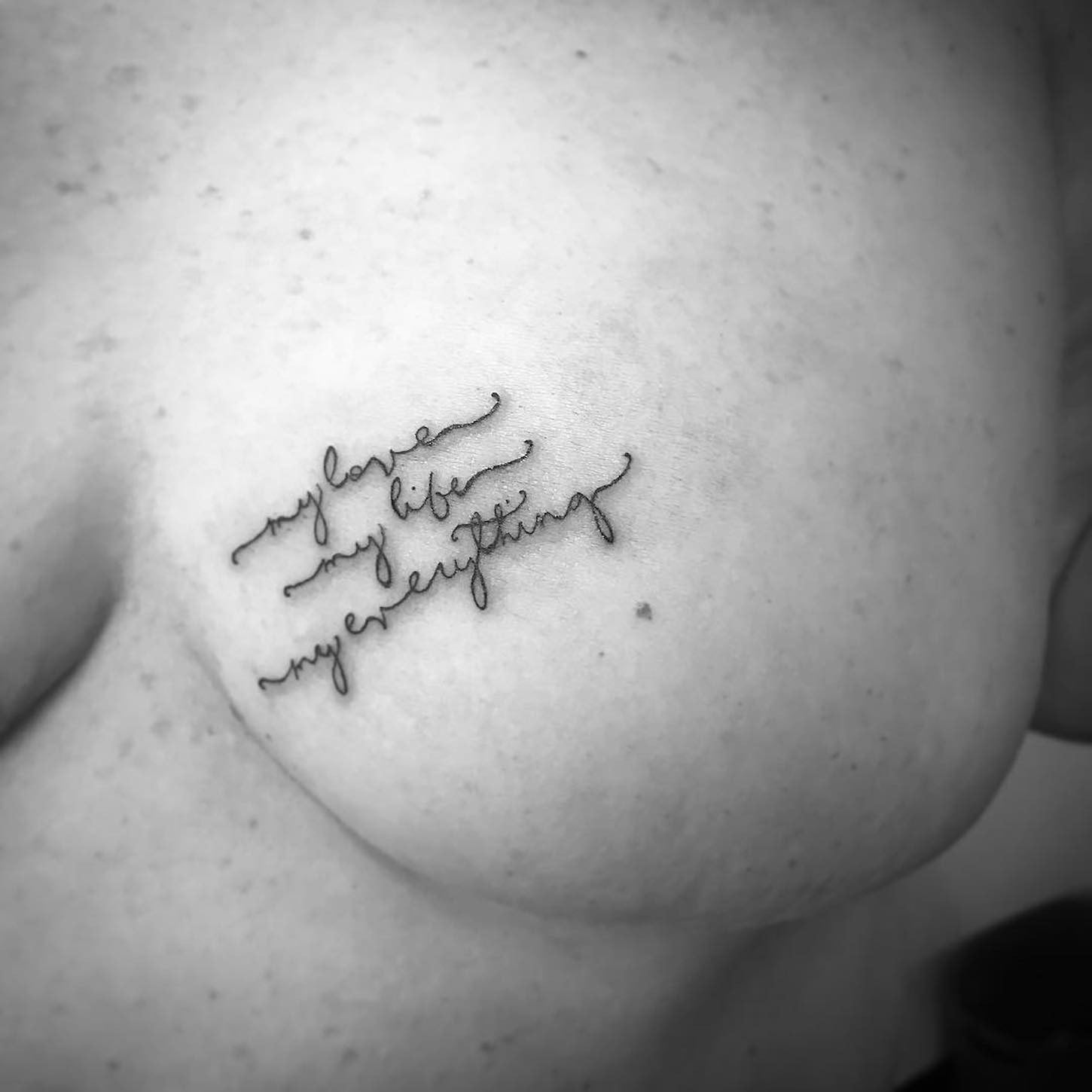This black and white professional photograph captures an intimate and powerful image of a woman's breast post-mastectomy, where one breast has been removed. The skin is freckled, displaying an array of small, dark spots scattered across a light grayish tone, typical of black and white photography. The focal point of the image is a delicate tattoo, written in elegant, thin black cursive lettering that reads, "my love, my life, my everything," arranged vertically in three centered lines. The text is slightly angled, adding a touch of grace to the composition. The photograph not only portrays physical resilience but also carries an emotional depth, symbolized by the meaningful and classy tattoo. In the lower right corner, there is a solid black area that frames the image and emphasizes the visual and emotional content.